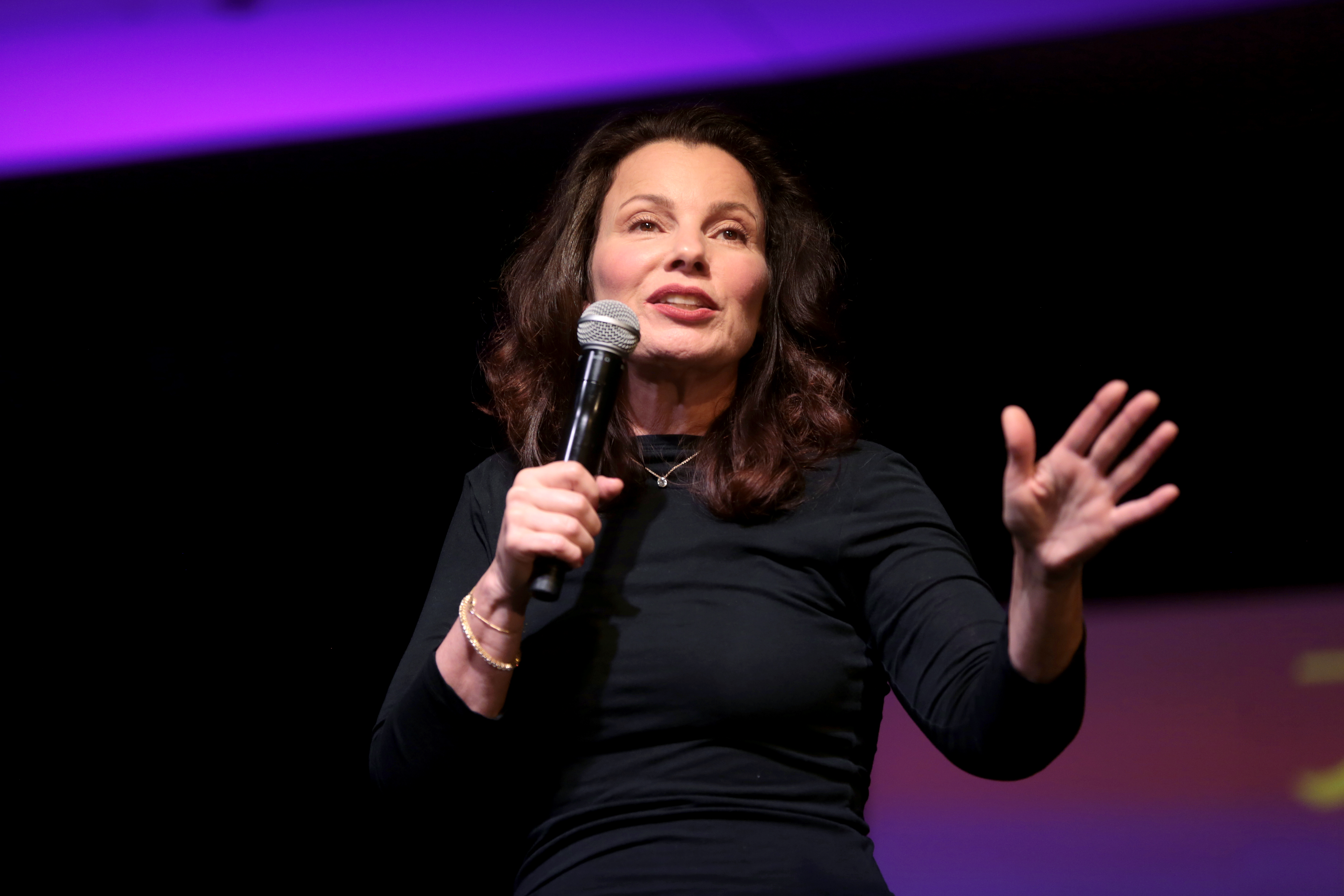The photograph captures Fran Drescher, a Caucasian woman with brown hair and light skin, likely in her late 50s, during what appears to be the Actors' Strike. She stands on a stage, in front of a predominantly black background that features striking neon purple and magenta stripes at the top and in the bottom right quadrant. Drescher, dressed in a long-sleeved black dress, is in mid-speech, holding a black microphone with a silver head in her right hand. Her left hand is outstretched in a gesturing manner towards the audience, emphasizing her point. She wears a noticeable pendant around her neck and a gold wristband on her left wrist, adding subtle touches of silver and gold to her ensemble. Her expressive face, framed by light wrinkles, is directed towards the crowd, signifying her engagement with the audience.